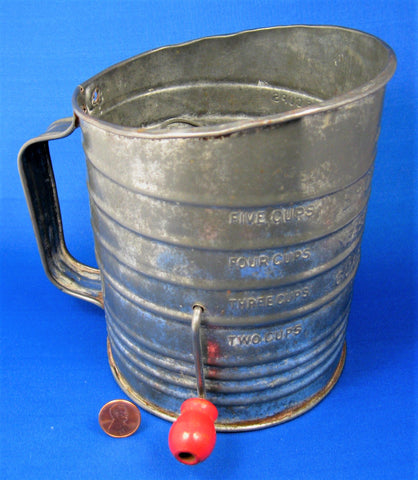This image, presented in a vertically aligned rectangular format, showcases an old-fashioned metal flour sifter set against a bright blue background. The sifter, likely made of silver material, occupies the center of the composition, revealing its well-used charm. A prominent handle extends from the left side, while on the right, the container widens slightly at the top, indicating the pouring spout. Etched into the metal are measurement lines that read "2 CUPS," "3 CUPS," "4 CUPS," and "5 CUPS" in capital letters from bottom to top. Across the middle, a red-handled crank protrudes from the sifter's side, used for sifting flour. Notably, a penny lies at the bottom left corner of the frame, underscoring the sifter's size. The base of this antique kitchen tool is tinged with rust, adding to its nostalgic appearance.